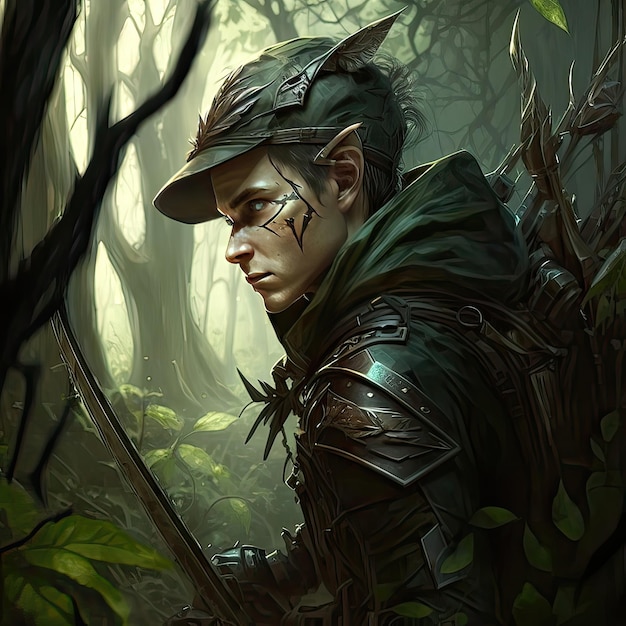In this digitally animated square image, the central focus is a young, fantasy-inspired archer warrior set against a lush, yet eerie woodland backdrop. The scene depicts barren trees devoid of leaves, with green shrubs, vines, and grasses contrasting the dark, misty atmosphere of the forest, possibly suggesting a swamp. Leaves are scattered across the ground, enhancing the mystical ambiance. 

In the foreground, the detailed image of the archer captures him from the elbows up, facing left. Clad in green and brown leather armor accented with metal plating on his shoulder, he personifies a classic fantasy archer. His attire includes a green jacket with a hood and a matching green cap adorned with wing-like extensions that mimic elf ears, adding to his enigmatic appearance. Although his ears are normal, an item attached to his ear further enhances the elf-like illusion.

This archer, carrying a bow and arrows along with a backpack that appears full of weapons, displays a tattoo or face paint running along the left side of his face and upper cheekbone. He strikes a composed yet vigilant pose, with a sword also visible among his gear, encapsulating the essence of a skilled and battle-ready hunter in a magical forest setting.